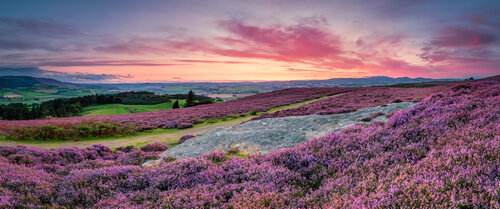The photograph showcases a breathtaking sunset landscape with a prominent rolling hillside in the foreground, blanketed by a field of lush purple wildflowers, possibly lavender. The flowers appear densely packed, creating a vibrant, continuous tapestry of color. Scattered patches of grass and a noticeable grey rock fragment add texture to the scene. Beyond the floral expanse, verdant green valleys and farmlands stretch out, bordered by lines of darker trees. The distant horizon features modest rolling hills and perhaps faint silhouettes of mountains. The sky, transitioning from a bright orange and yellow near the horizon to a soft pink and finally a deepening blue, is speckled with wispy cirrus clouds that take on a purple hue as they drift above. The vivid colors underscore the beauty of the setting or rising sun just below the horizon, lending a magical ambiance to the entire landscape.